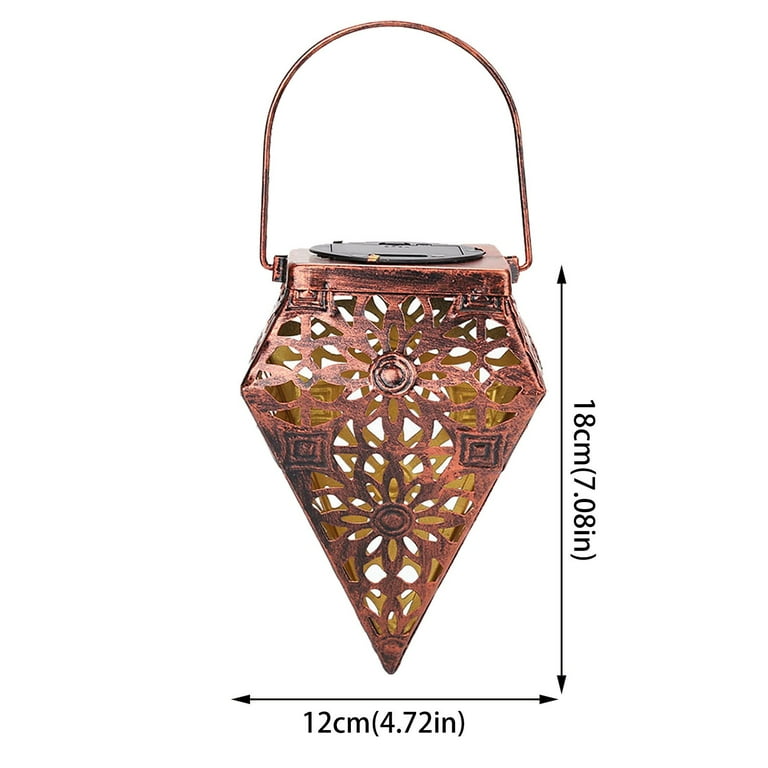This photographic image depicts an ornate, copper-colored lantern floating against a white background, devoid of any setting. The lantern has an inverted triangular shape with a metal handle on top, attached to a small black lid that appears to slide off for placing items inside. The design features intricate cutouts, including flower petal motifs and circular patterns at the center, complemented by square designs on the sides. The transparency of the metal allows a clear view of the interior. Measurement lines with arrows indicate its dimensions: 12 centimeters (4.72 inches) in width and 18 centimeters (7.08 inches) in height.